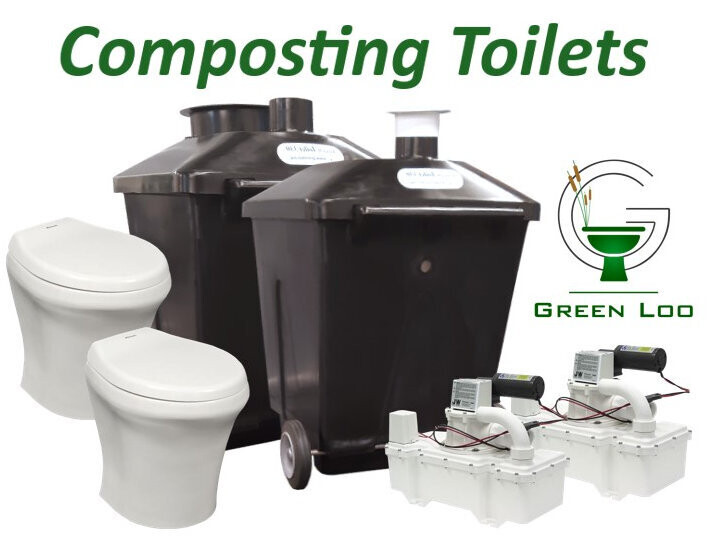**Advertisement: GreenLoo Composting Toilets**

---
Transform your approach to waste management with GreenLoo Composting Toilets. In our ad, prominently featured is our brand logo—a stylized green toilet bowl with an artistic touch of pussy willows where the seat back would be, all enveloped by a dynamic double 'G'. 

Our comprehensive composting solution includes a set of two of each essential component for a complete installation. Featured are:
- Two sleek, white toilet seats designed for comfort and efficiency.
- Two robust black tanks, one with visible wheels for easy mobility, tasked with processing your composting matter.
- Two advanced motors engineered to ensure optimal operation and odor control.

Elevate your eco-friendly options with GreenLoo, where our innovative design meets practicality.